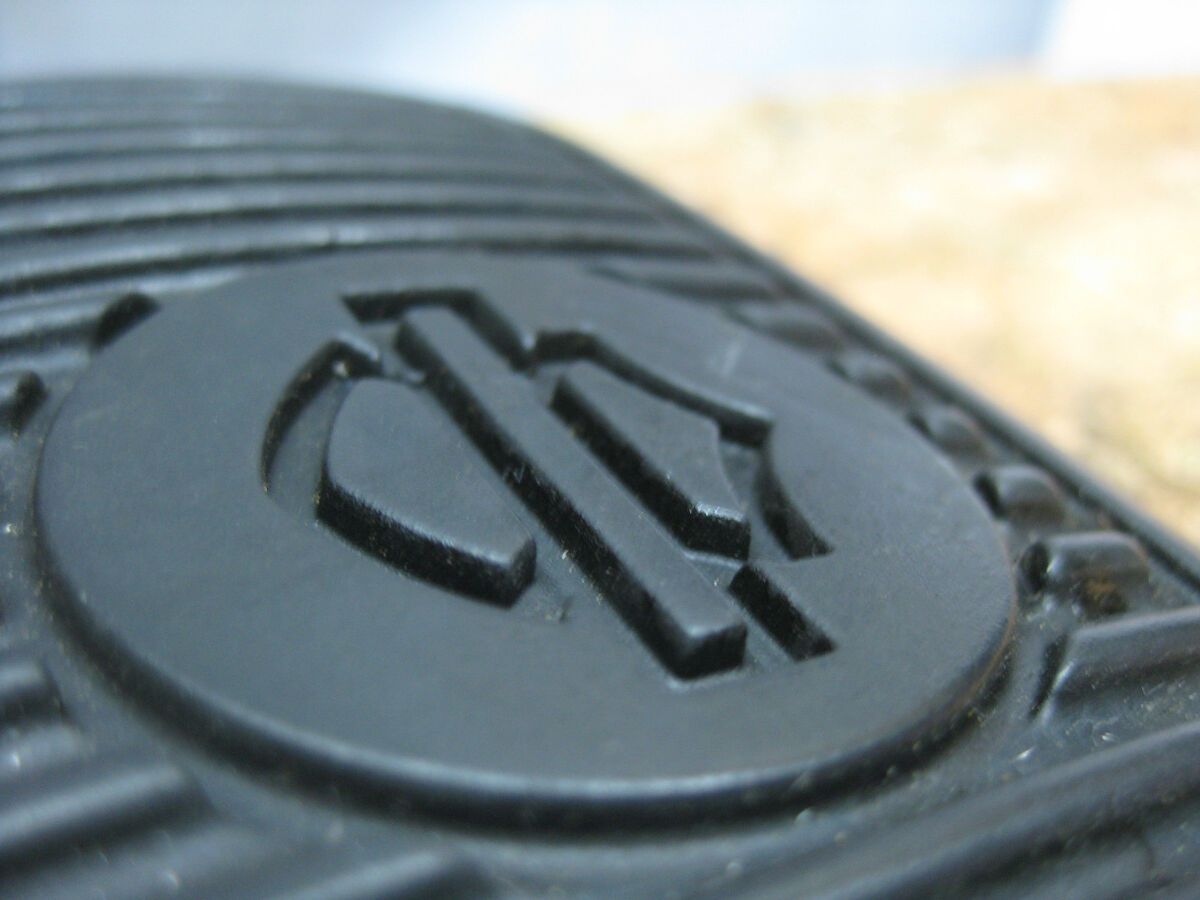This detailed image appears to showcase a close-up of a dark gray or black grill element, possibly part of a Harley-Davidson logo or similar design. In the bottom left, there's a prominent round section featuring a sunken, tall rectangular shape with wing-like extensions on each side. This design is flanked by grooves that resemble those found on an indoor grill. In the top right corner, a cream-colored surface is visible, with the sky serving as the backdrop, adding depth and contrast to the composition.